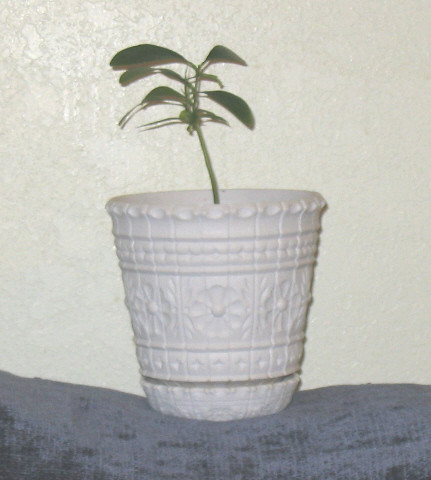The image features a minimalistic and simple scene of a young houseplant in a white vase, situated on a blue blanket which appears to be covering a soft, fabric-like surface. The setting suggests the plant may be resting on a couch or bed, given the indentations visible in the blanket, which is a purpley-blue with gray-black splotches. The white vase is detailed with horizontal light gray lines, a fluted edge at the top, and a dark demarcation near the bottom where it narrows. The plant itself is small with a single green stem approximately eight inches tall, from which a few leaves branch out. The backdrop is a very white wall with some cream undertones, casting shadows of the plant's leaves. The overall ambiance suggests that the plant might be suited to a low-light environment inside the home.